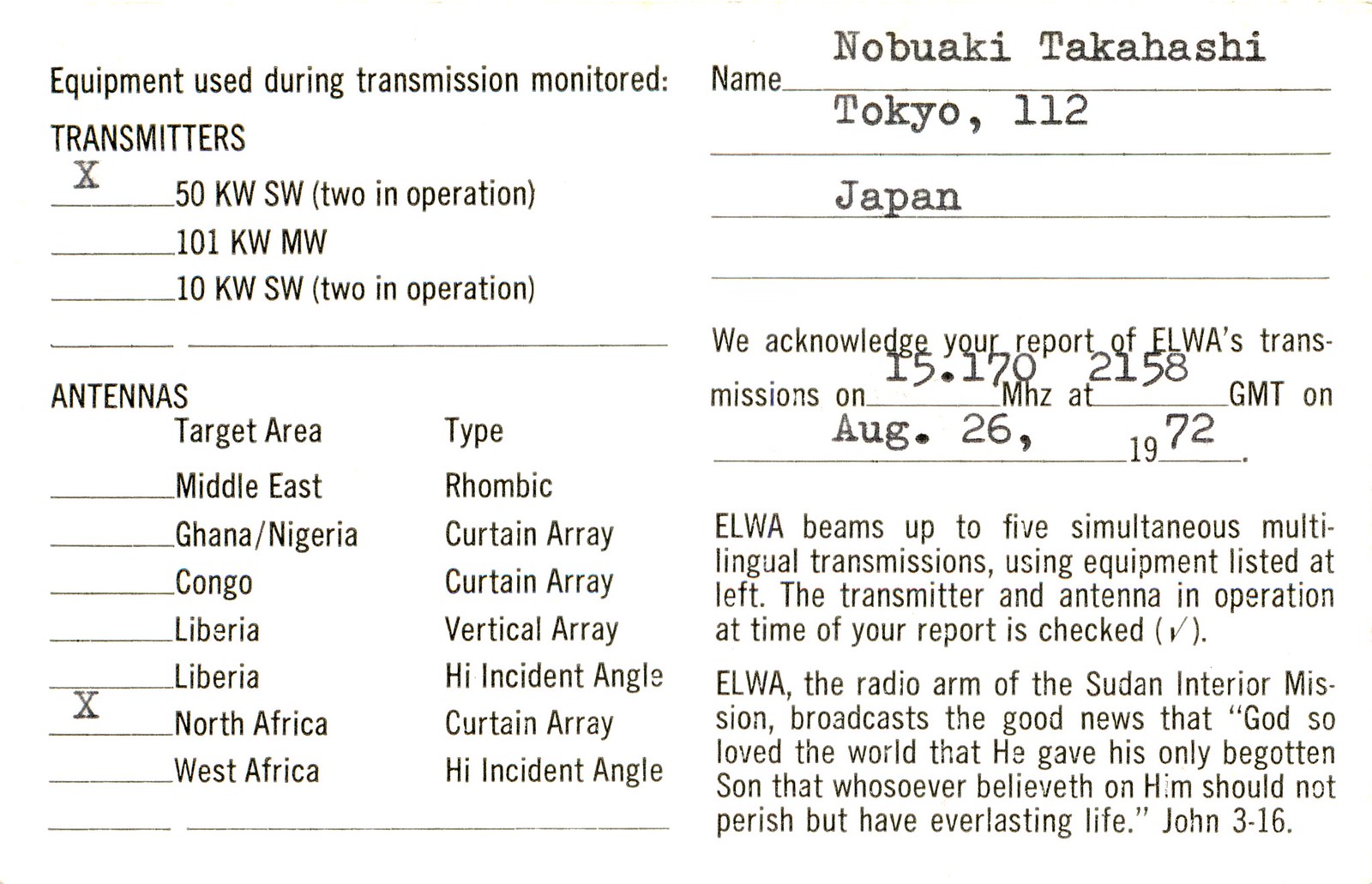The document displayed features a structured layout, primarily divided into a left-hand and right-hand section. On the left-hand side, there's a heading that reads "Equipment Used During Transmission Monitored," followed by the subheading "TRANSMITTERS" in all capital letters. Below this header, there are three specific transmitter options listed:

1. "50 kW SW in operation" (with an X marked next to it),
2. "101 kW MW," 
3. "10 kW SW in operation."

In the right-hand section, beneath the heading "Name," there are four lines. The first line extends directly from the word "Name," followed by three additional lines underneath. The name "Nobaki Takahashi" is typed out on these lines. Below the name, "Tokyo, 112" is mentioned, followed by "Japan."

Returning to the left-hand side, just below the "Equipment Used During Transmission Monitored" heading and the "TRANSMITTERS" list, there is another section titled "ANTENNAS." Here, various options are listed, with an X marked directly on "North Africa."

On the right-hand side, below the "Name" section, there is a statement acknowledging the report: "We acknowledge a report of Elwa's transmission on 15.17 megahertz at 215 A GMT on August 26, 1972," followed by additional related information.

Overall, the document meticulously records specified equipment, locations, and corresponding acknowledgments related to the monitored transmissions.